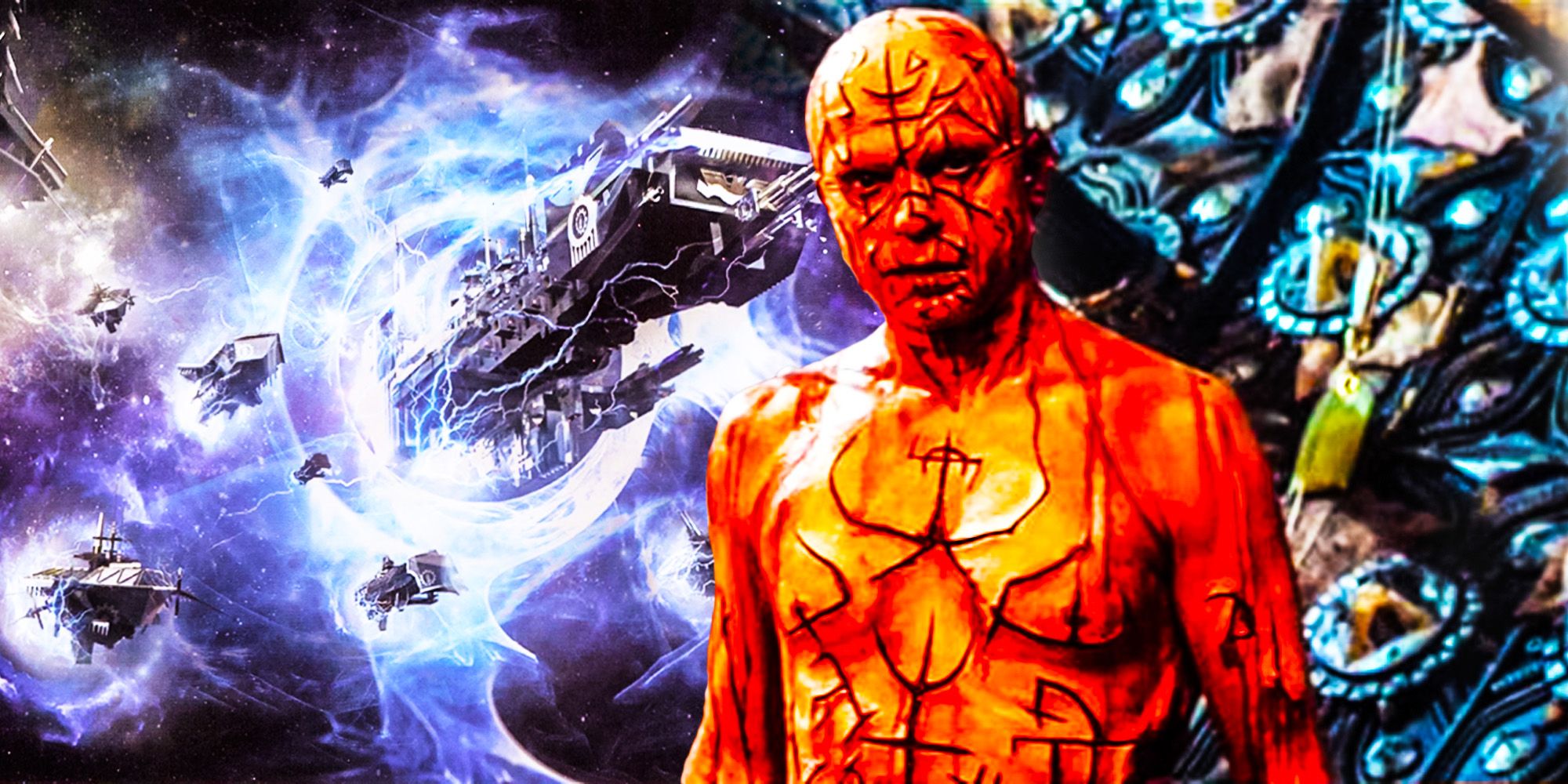In the foreground of this detailed digital drawing, an imposing, bald male figure stands, his entire body awash in vivid oranges and reds. His flesh is adorned with intricate, symbolic carvings or scars that give the appearance of dark hieroglyphs and demonic representation, with some areas tinged in blood and dark ichor. His eyes, nose, and mouth are distinctly visible, and he exudes a sinister, almost devilish aura, enhanced by the raised, orange skin around the etched markings. His expression is one of severe determination. His torso is decorated with bright yellow patterns that resemble flames, with a prominent cross-like symbol featuring a half-circle and extending lines.

Behind this unearthly figure, an ethereal vista opens up to the vastness of space. To the left, several colossal, alien-looking spacecraft emerge from a tumultuous electrical storm or hyperspace. These ships, rendered in dark silver and black, appear to be caught in an electromagnetic field radiating electric plasma, creating an impression of chaos and otherworldly power. Blue and yellow stained glass and multiple TV screens or perhaps floating monitors can be seen among the swirling backdrop of electric blue energy, adding to the surreal and futuristic ambiance of the scene.